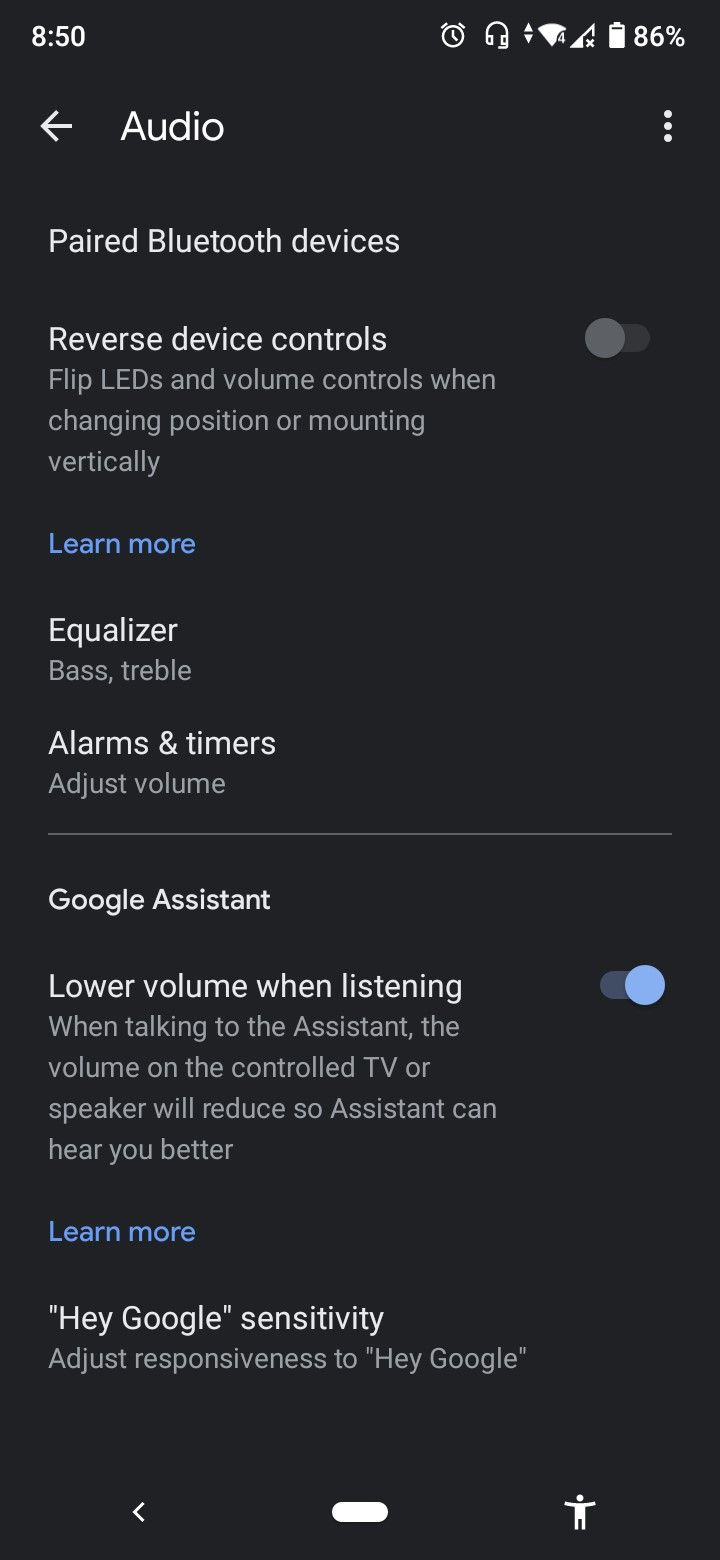The image showcases a smartphone screen displaying a settings menu with a sleek black background. In the top left corner, the time is indicated as 8:50, and the battery is at 86%. An arrow pointing to the left accompanies the label "Audio..." Immediately below, the section "Paired Bluetooth Devices" is visible.

Continuing down the screen, the "Reverse Device Controls" option is mentioned with specific instructions: "Flip LEDs and volume controls when changing position or mounting vertically," which is currently toggled off, indicated by a button that can be switched on. A "Learn More" link in blue is available for further information.

Further, the "Equalizer" section lists options for adjusting "Bass" and "Treble." Below this, the "Alarms and Timers" section is detailed, including an "Adjust Volume" option. A faint gray line spans across the screen, delineating different sections.

The lower portion of the screen introduces the "Google Assistant" section, where the option "Lower volume when listening" is turned on. At the very bottom, the "Hey Google Sensitivity" setting is mentioned, allowing users to adjust the responsiveness to the "Hey Google" command.